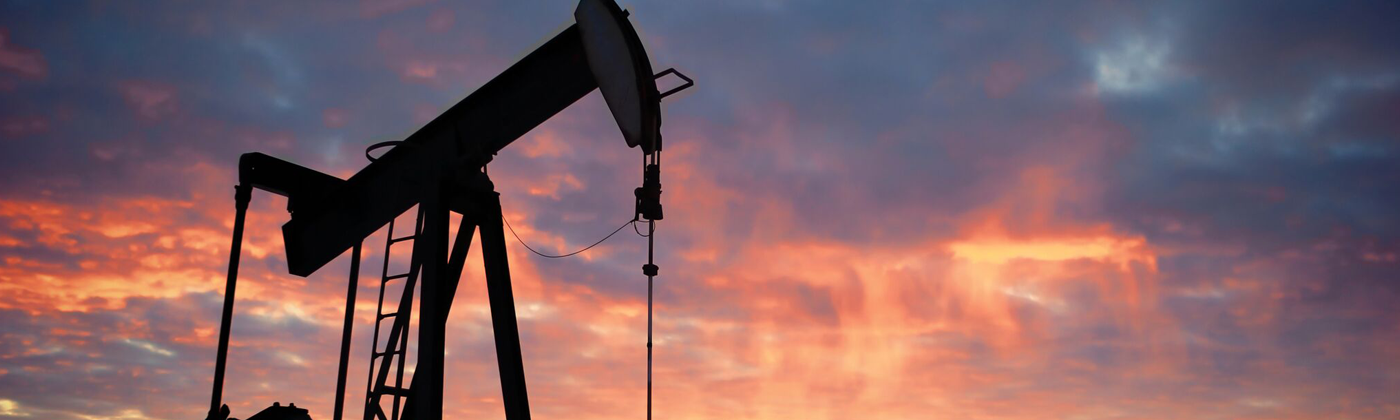In the foreground of this photograph stands a silhouetted oil rig, its dark outline blending almost seamlessly with the evening sky. The rig appears predominantly black, with a faint touch of white at the end, presumably where it dips toward the ground. The setting is twilight, characterized by a stunning and vibrant display of colors as the sun sets. The sky is filled with an array of clouds, ranging from blue to orange-pink hues, with the latter becoming more pronounced toward the right side of the image. These colors, a mix of orange, red, and pink, create a dramatic and beautiful backdrop that accentuates the scene's atmospheric beauty. The ground is not visible in the photograph, ensuring the viewer's focus remains on the interplay between the silhouetted rig and the striking evening sky.